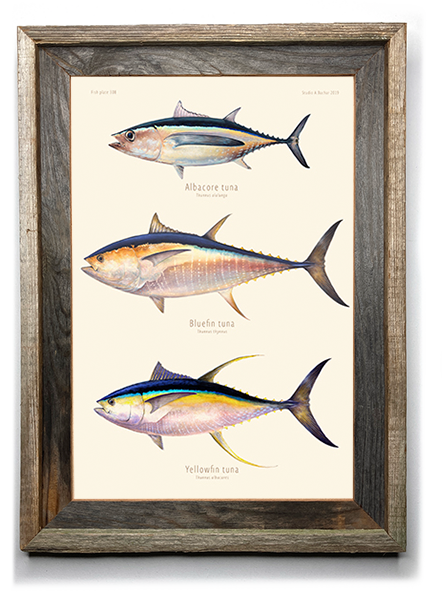The photograph depicts a wall hanging framed by a medium brown wooden border with beige and tan stripes. Inside this frame, there is another, darker wooden trim that encloses a white background showcasing three colorful fish drawings stacked vertically. Each fish's mouth faces the left, and their tails point to the right. At the top is the smallest fish, labeled "albacore tuna," featuring a blue stripe near the top of its body, with subtle bluish, yellowish shimmers below it, and a predominantly white body with darker shades on its fins. The middle fish, identified as "bluefin tuna," is the largest, characterized by a similar blue stripe, orange and white hues on its sides, and a more prominent white belly. The bottom fish, marked as "yellowfin tuna," displays a blue stripe with lighter blue and yellow beneath it, along with a white belly area. Additional text is present at the top left and right corners of the drawing, though it is not legible in the image.